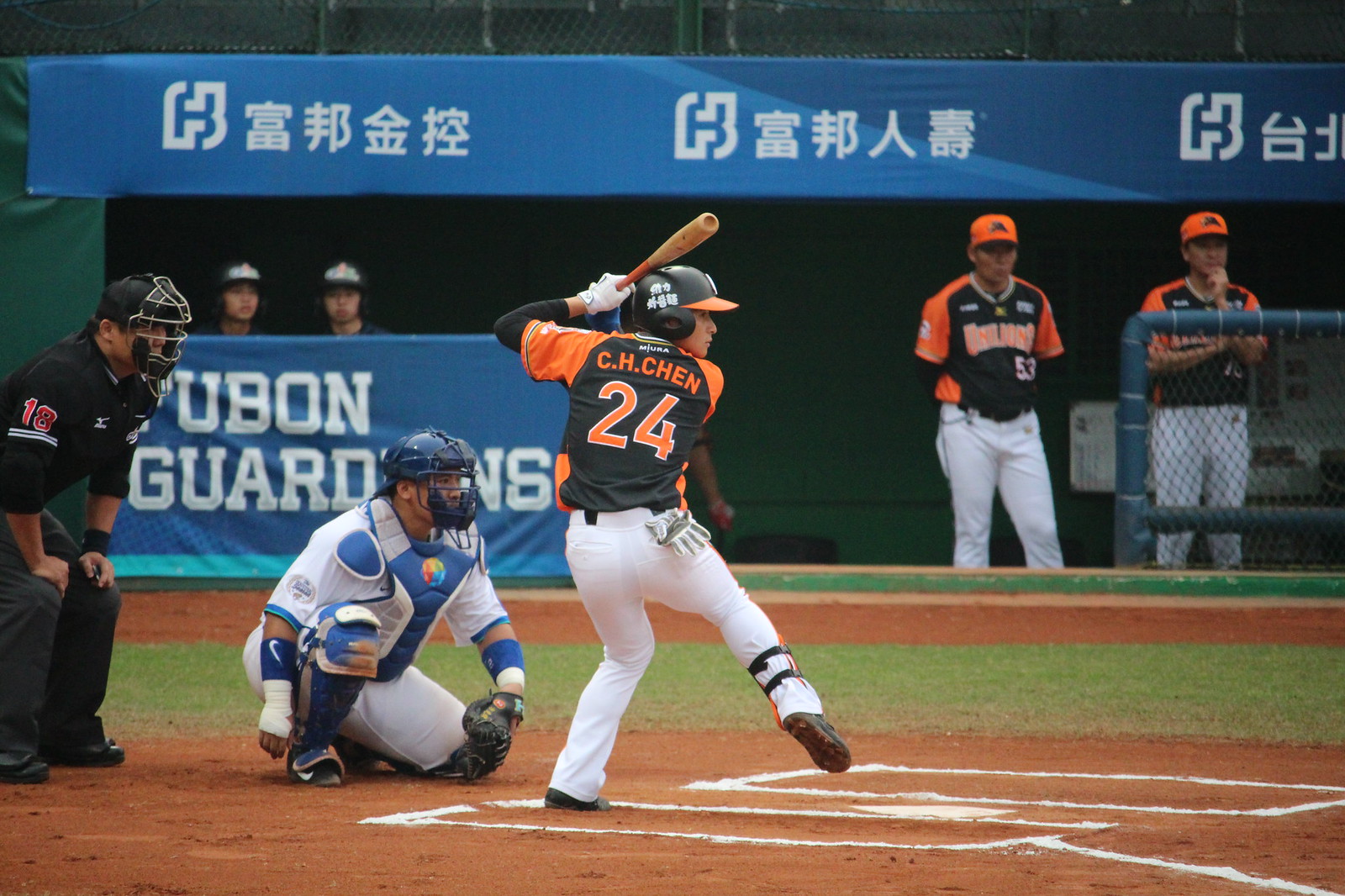In this detailed photograph of a baseball game, likely set in an Asian country as suggested by the blue banner with white Chinese characters in the background, the focus is on a baseball player preparing to bat. The central player, donning a black and yellow jersey with "C.H. Chan 24" printed on the back, white pants, and an orange cap, is poised to swing, with one arm pulled back and a determined stance, balancing on one foot. Directly behind this batter, the catcher, dressed in a white and blue jersey, a brown helmet, and a blue caged mask, is kneeling on the ground, ready to receive the pitch with a black mitt. Positioned further behind the catcher is the umpire, dressed entirely in black, including a caged helmet, and bending over with his hands on his knees. To the left of the image, another player in a black jersey is squatting, observing the scene closely. The dirt of the home plate and the vibrant green grass of the field are clearly visible, enhancing the game's dynamic atmosphere, while several other players watch intently from the dugout area.